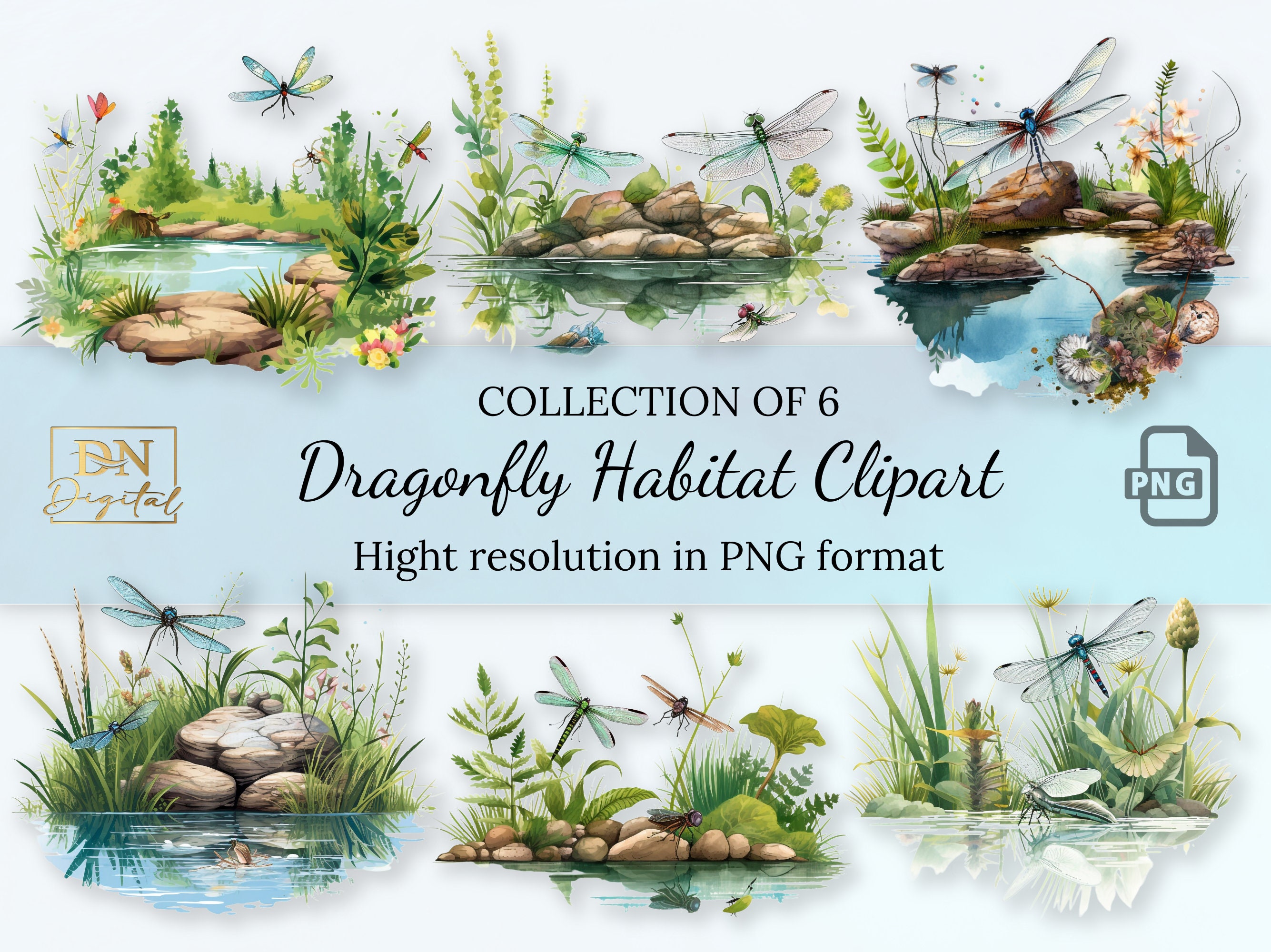The promotional banner is a rectangular digital poster designed to showcase a downloadable or purchasable set of six high-resolution dragonfly habitat clip art images in PNG format. The banner's layout features three distinct sections with a prominent focus on dragonfly-themed artwork. 

The background is divided into three horizontal sections. The top and bottom sections, both sporting a light blue background, display three dragonfly-related illustrations each. These drawn illustrations, reminiscent of children's book art, depict serene dragonfly habitats characterized by water bodies, stones, and lush green vegetation. The dragonflies, with their bright-colored bodies and translucent, multi-hued wings, can be seen flying gracefully around the scenes, adding to the picturesque quality. Additionally, other animals like horses and grasshoppers appear in the illustrations, further enriching the natural settings.

The center section consists of a solid blue horizontal strip that runs across the width of the banner. On the left side of this strip is a gold square logo with the text "DN Digital" inside it. Centrally positioned within the strip is a bold, black printed text that reads: "Collection of Six Dragonfly Habitat Clip Art High Resolution in PNG Format." On the far right of the strip, there is an icon resembling a rectangular piece of paper with the label "PNG" on it, representing the format of the clip art files available. This cohesive arrangement effectively highlights the detailed and vibrant dragonfly illustrations while providing essential information about the digital collection.